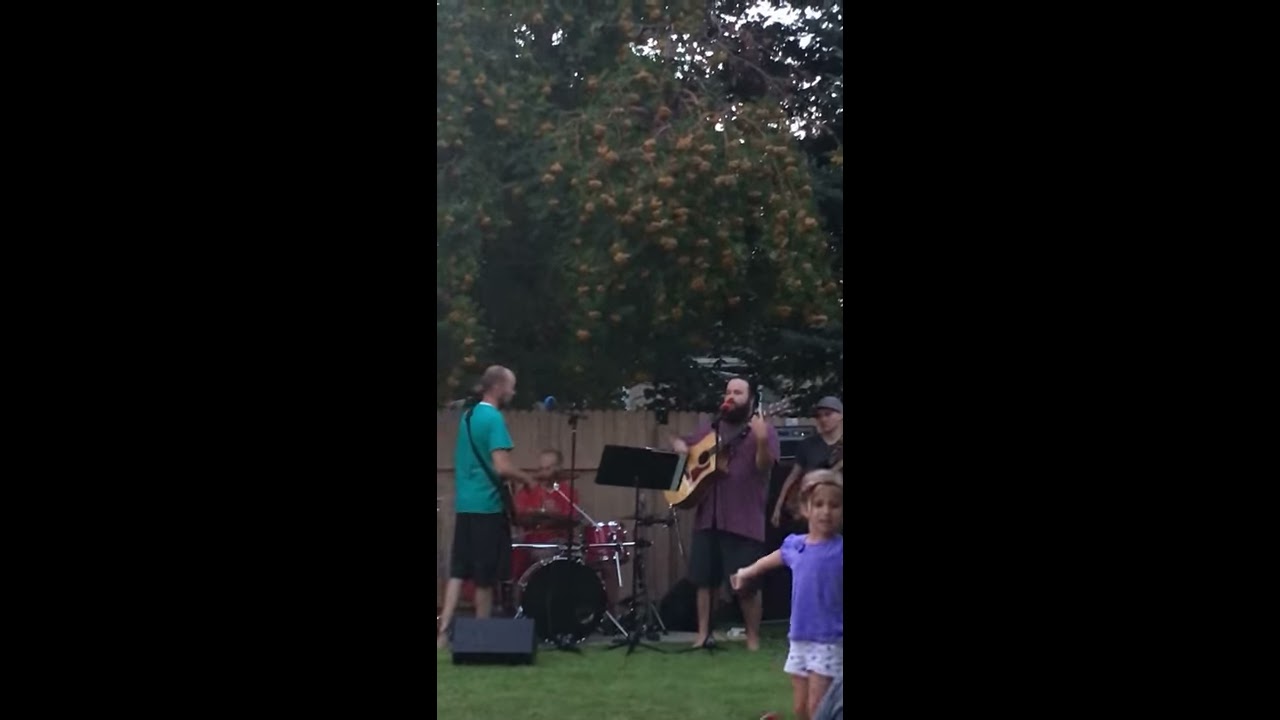In this vivid outdoor scene, a casual musical band is positioned on a lush, green lawn bordered by a tall wooden privacy fence. The group comprises five individuals. Furthest to the left stands a man in a short-sleeved teal shirt and black shorts, distinguished by a short-cropped hairstyle and a receding hairline. A strap runs diagonally across his shoulder. Next to him, partially obscured, is a man seated at a drum set with a prominent black bass drum, clad in a red shirt. Central to the scene is a bearded man with a dark complexion, sporting a rune-colored, short-sleeved button-up shirt and black shorts. He cradles an acoustic guitar with a wooden body and a red pickguard. To the right, another young man in a black shirt and gray cap directs his gaze towards an unseen audience, possibly signaling his involvement in the performance. 

In the foreground, a young girl with her back to the scene dons a purple shirt and white shorts. She extends her arm outward, adding an element of motion and liveliness to the image. Scattered on the ground in front of the ensemble are black amplifiers, hinting at their musical setup. Towering behind the wooden fence stands a large, dense tree brimming with green leaves, its heavy branches drooping slightly, contributing to the picturesque and serene backdrop.